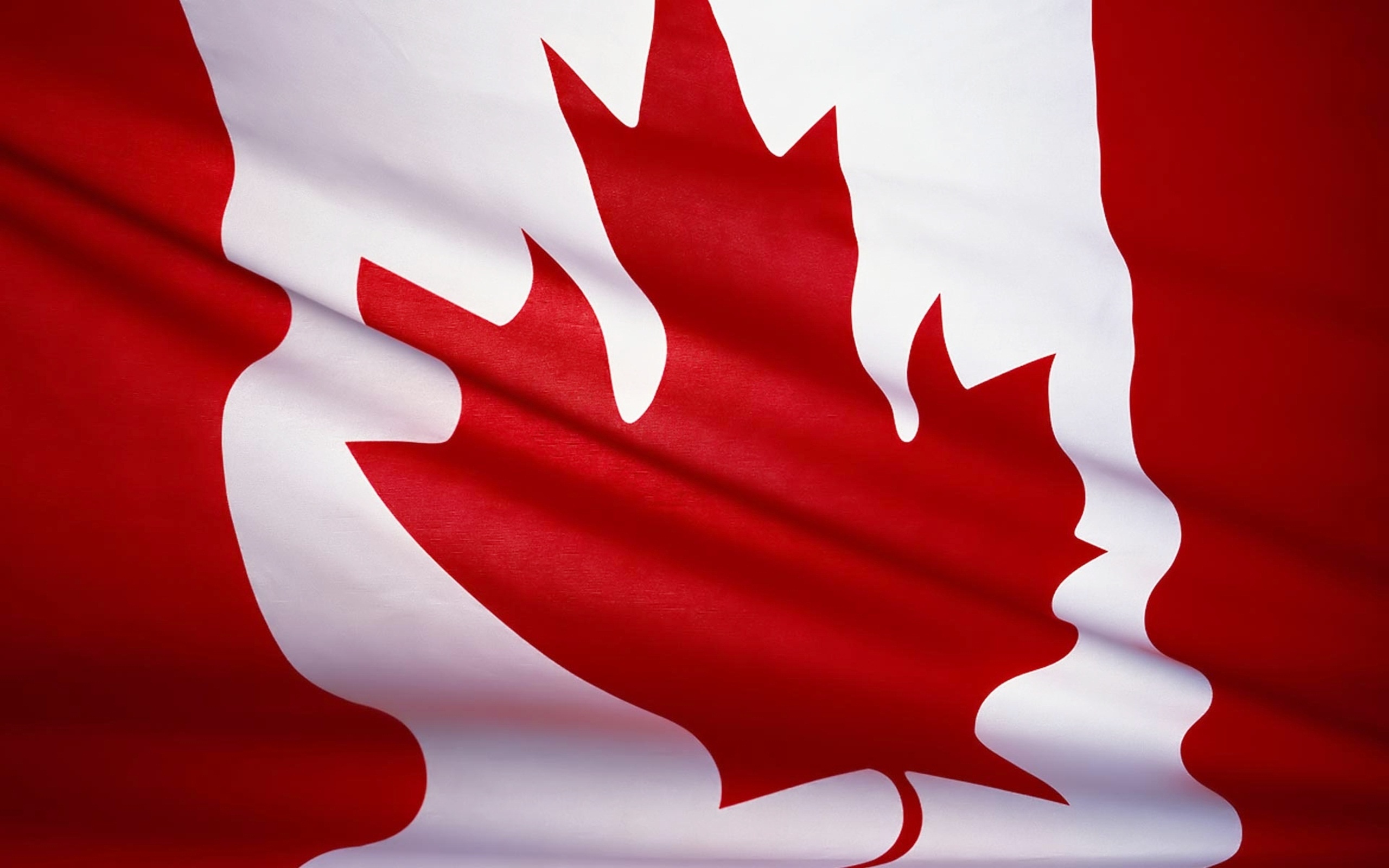The image features a close-up of a slightly wrinkled Canadian flag. Central to the composition is a prominent red maple leaf set against a white background, with solid red vertical sections on both the left and right sides. The maple leaf, positioned directly in the middle, extends from the top to the bottom of the visible area, with its stem slightly bent as if the flag is folded or caught in a breeze. Notably, there is a prominent diagonal fold running from near the top left corner down to the bottom right, creating additional creases that make the edges of the red and white sections appear wavy. The flag fills the entire frame, emphasizing its folds and texture.